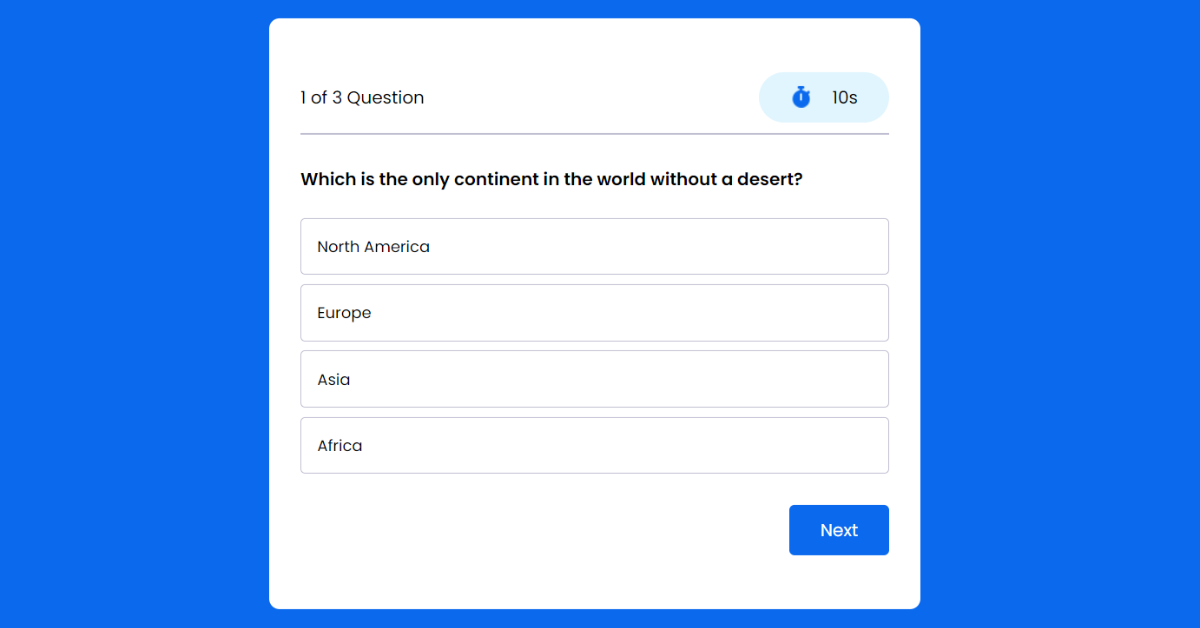The image features a bright blue background with a central square approximately six inches in length. To the left of the square, there is text that reads "One of Three Questions" alongside two circles—one in blue and the other in a darker blue. The darker blue circle contains a clock symbol indicating "10 seconds."

Below this, in black text, is a question: "Which is the only continent in the world without a desert?" The multiple-choice options that follow the question are: North America, Europe, Asia, and Africa. At the bottom of the image, there is a blue rectangular button approximately two inches long with the word "Next" inside it, intended for users to click and proceed.

The overall design emphasizes the quiz-like nature of the content, focusing viewers on the task of identifying which continent lacks a desert. The clarity of the options ensures that viewers understand their choices, with the names of the continents clearly spelled out: North America, Europe, Asia (A-S-I-A), and Africa (A-F-R-I-C-A).